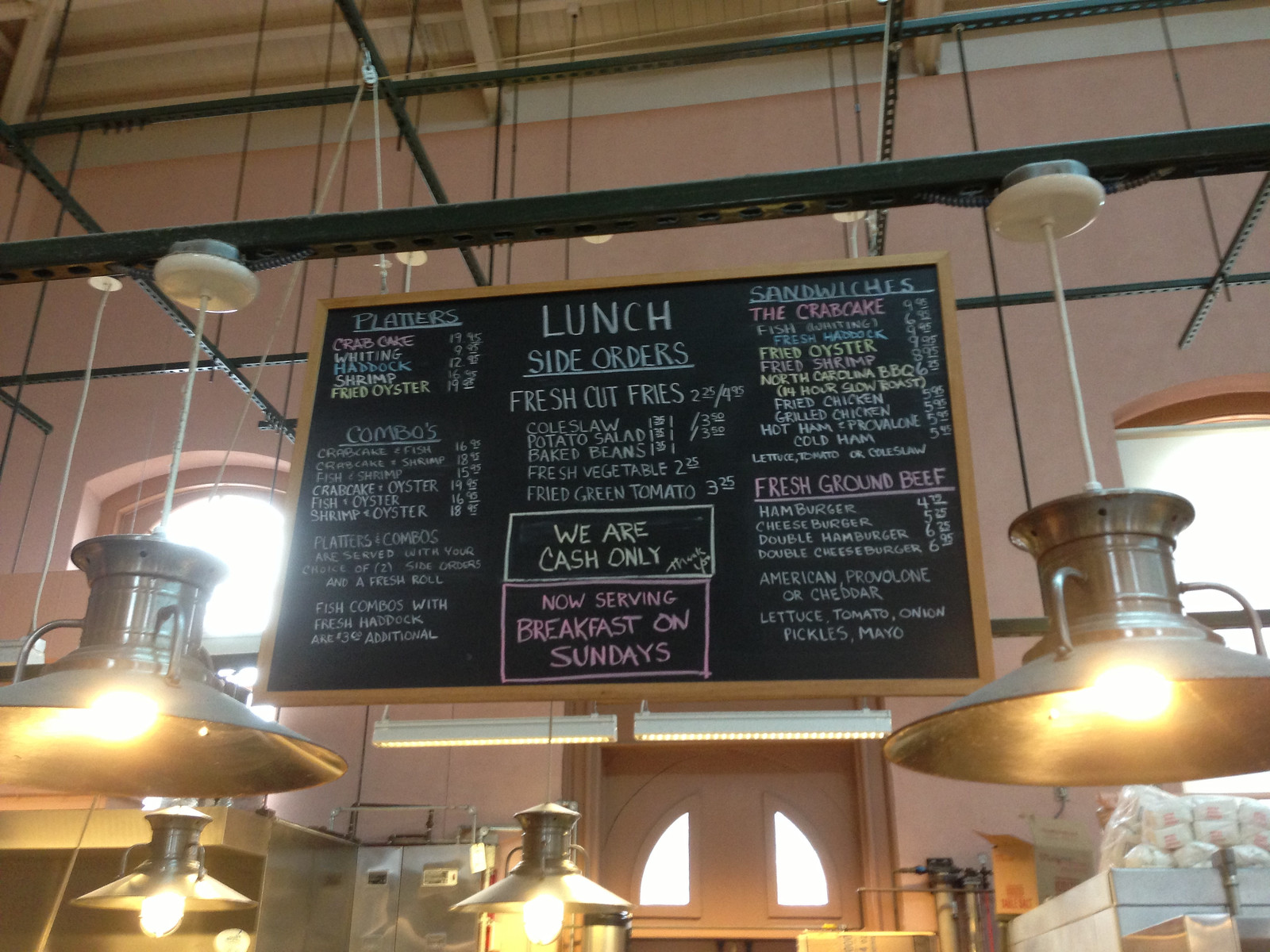The photo depicts a chalkboard menu at a restaurant, suspended from the ceiling with visible metal bowl lights, illuminating the board without any coverings. The blackboard, encased in a wooden frame, features the menu in colorful chalk.

At the top center, a light blue "Lunch" heading is prominently displayed. On the left side, under "Platters," options like crab cake, whiting, haddock, shrimp, and fried oysters are listed, followed by "Combos" such as fish and oysters or fish and shrimp, with prices indicated. A note mentions that all platters and combos are served with two side orders and a fresh roll, and specifies an additional $3 charge for fish combos with fresh haddock.

In the middle section, under the "Side Orders" heading, sides such as fresh-cut fries, coleslaw, potato salad, baked beans, fresh vegetables, and fried green tomatoes are detailed along with their prices. Below this, a yellow chalk note states "We are cash only, thank you." Further down, in pink, the board announces, "Now serving breakfast on Sundays."

On the right side, the "Sandwiches" section includes options like crab cakes, fried oysters, fried shrimp, North Carolina BBQ, fried chicken, grilled chicken, hot ham and provolone, and cold ham. This section is followed by a list of "Fresh Ground Beef" choices, including hamburger, cheeseburger, double hamburger, and double cheeseburger, with additional details like cheese options (American, provolone, or cheddar), and condiments (lettuce, tomato, onion, pickles, mayo).

The overall ambiance suggested by the lights and the daytime window lightings in the background, conveys a bright and inviting atmosphere in the restaurant.